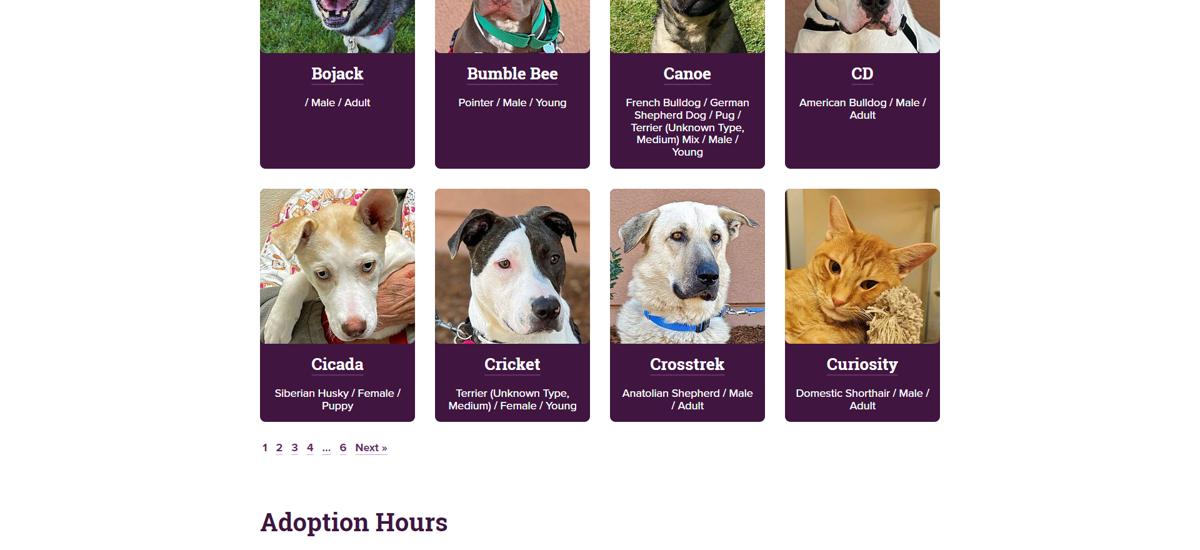The website features a user interface that exudes a minimalistic aesthetic, reminiscent of mobile design despite being tailored for desktop. The homepage is segmented into tabs or panels showcasing a plethora of adoptable animals, predominantly cats and dogs. In the bottom left corner, there's a section labeled "Adoption Hours," indicating the specific times when adoptions can take place.

The panels prominently display a variety of animals, each with a photograph, although some images are partially cropped. Among the notable names, we find Bojack, Bumblebee, Canoe, Seedy, Cicada, Cricket, Crosstrek, and Curiosity. Curiosity is identified as a Domestic Short Hair cat, male and adult, standing out as the sole feline amid a sea of canines.

The majority of the animals listed are adult dogs, and gender representation skews heavily towards males, with only one clearly marked female animal. At the footer of the page, an indicator shows multiple pages—at least six more—filled with additional pets available for adoption, hinting at the extensive array of animals awaiting new homes.